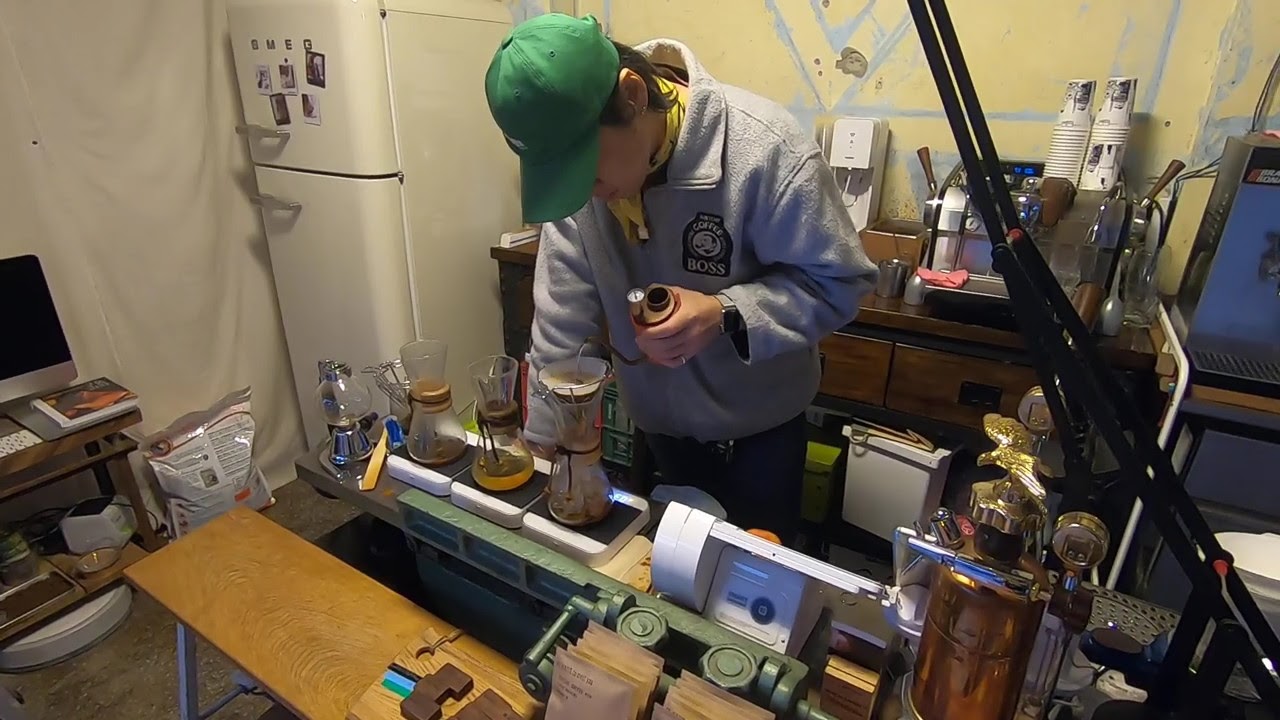The photograph is a detailed interior shot of a makeshift workshop or possibly a chemistry lab, taken in landscape orientation. The setting features a diverse mix of elements suggesting both a utilitarian and experimental atmosphere. On the left side of the image, a white older-style refrigerator stands with its freezer on top, adorned with horizontal silver handles, which lends an aged feel. Adjacent to the fridge is a computer table with a monitor and other computer equipment. The left side background is veiled with a white sheet, giving the setting a provisional look.

In the center of the scene is a young man, around 20 years old, wearing a green ball cap and a gray collared overcoat with an indistinct logo on the front left. He is bent over a sturdy table, which might have originated as a lathe or sawing table but now holds an array of scientific-looking apparatus. The table features three beakers with conical funnels on top, containing different colored mixtures. The young man appears focused on adding something to the beakers, holding items in his left hand.

To the right of the image, partially in the background, is a yellow wall. Directly behind the young man stands a machine that resembles either an ice cream or coffee machine, complete with stacks of paper cups on top. The background also includes a countertop with miscellaneous packages and kitchen utensils, contributing to the eclectic nature of the space. Additionally, there is a shredder placed somewhere behind the young man, further adding to the sense of functional chaos. The overall photographic style is representational realism, vividly capturing the blend of industrial, scientific, and everyday elements.